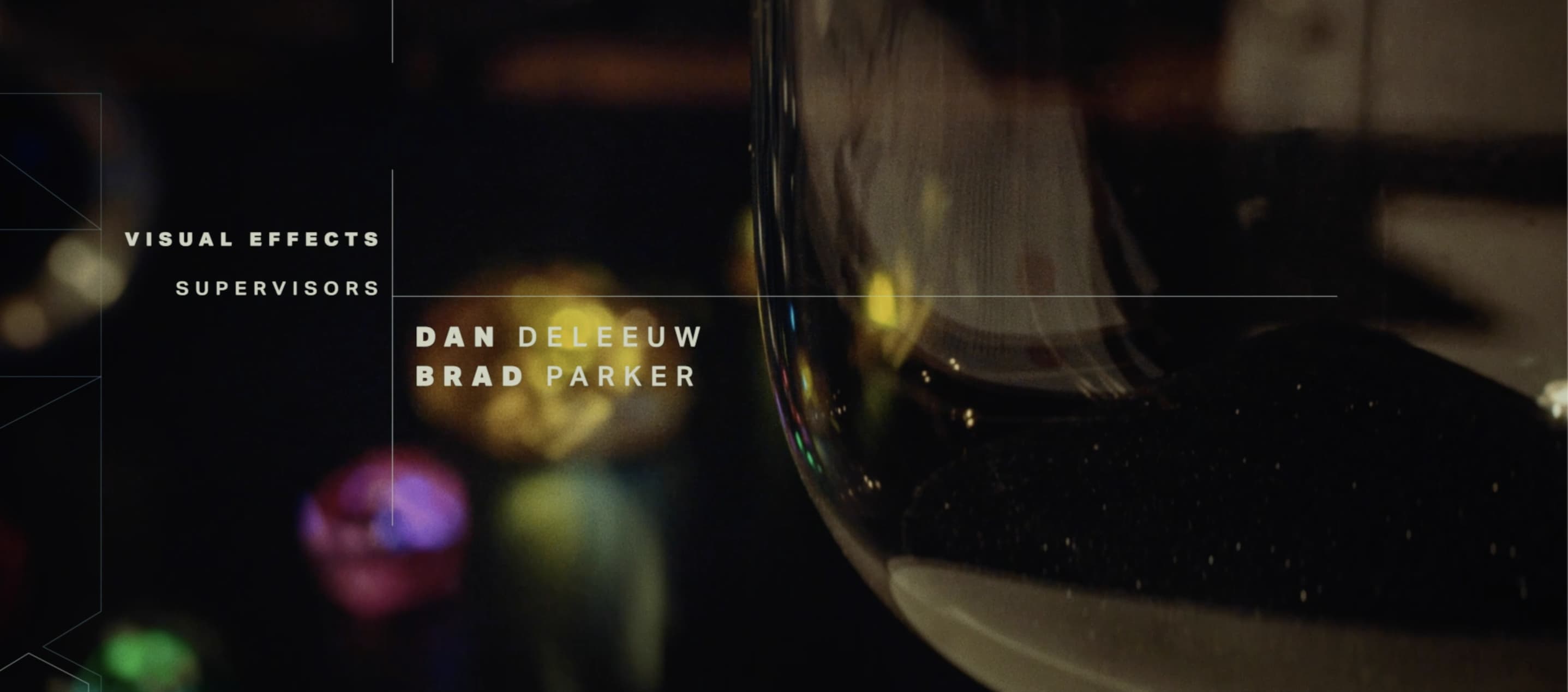The image captures a widescreen view reminiscent of movie end credits, with the title “Visual Effects Supervisors” prominently displayed in crisp white text on the left side of the screen. The names Dan DeLieu and Brad Parker are listed just to the right, slightly off-center. The background is predominantly black, featuring a series of blurred circles and spheres in various colors: pink, yellow, green, and a hint of purple. These spheres could be interpreted as bubbles or out-of-focus lights, adding a mysterious and abstract element to the scene. Dominating the right side is a dark sphere with a light reflection, potentially resembling a wine glass filled with dark red wine. This central object is surrounded by other spheres and circles, contributing to the image's overall abstract and cinematic quality.